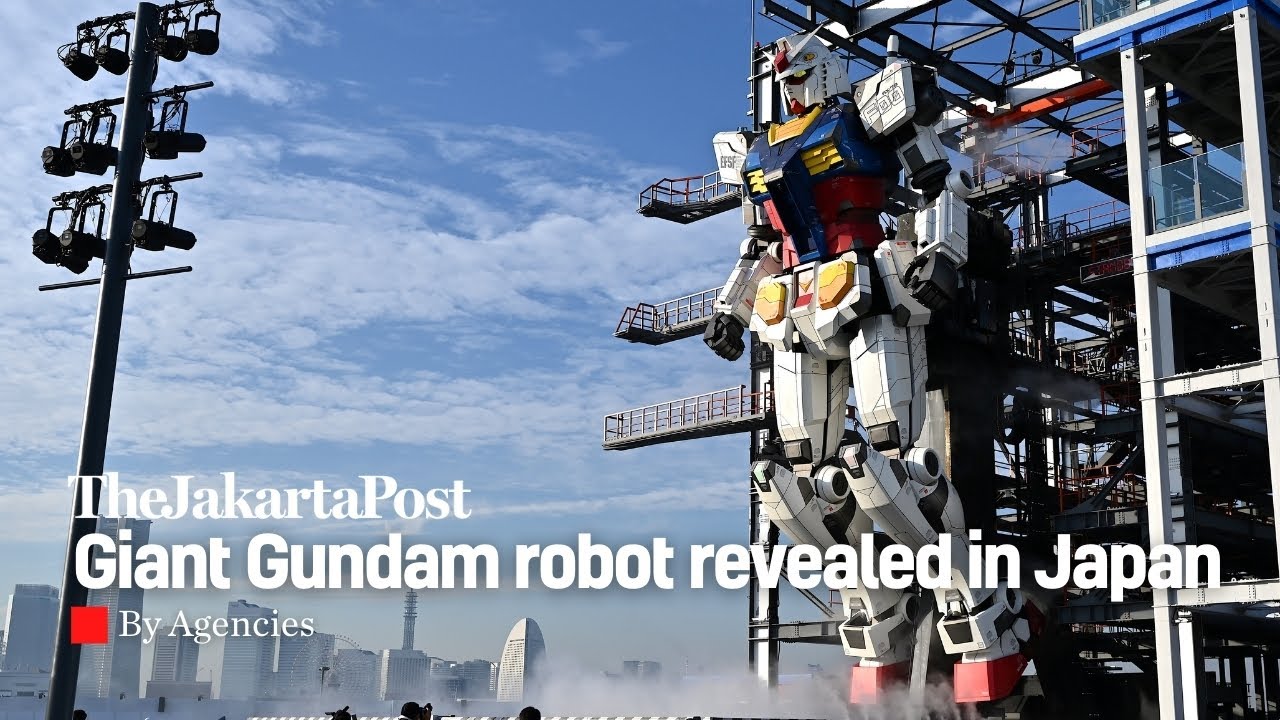The front page of a magazine from the Jakarta Post features the headline "Giant Gundam Robot Revealed in Japan" by Agencies. The photograph showcases a giant Gundam robot, reminiscent of a Transformer, being supported by an intricate scaffolding structure. The robot is prominently white, with notable blue and red sections on its chest and sprinkles of red and yellow accents across its body. The scaffolding, which is primarily white with red and blue elements, includes stadium-style lights to the left, possibly to illuminate the robot at night. In the background, a vast city skyline stretches beneath a light blue sky adorned with wispy cumulus clouds. Text on the image is all in white, and next to the words "By Agencies" is a small red square. Balconies are visible coming off the scaffolding, and a boardwalk can be seen above the robot.